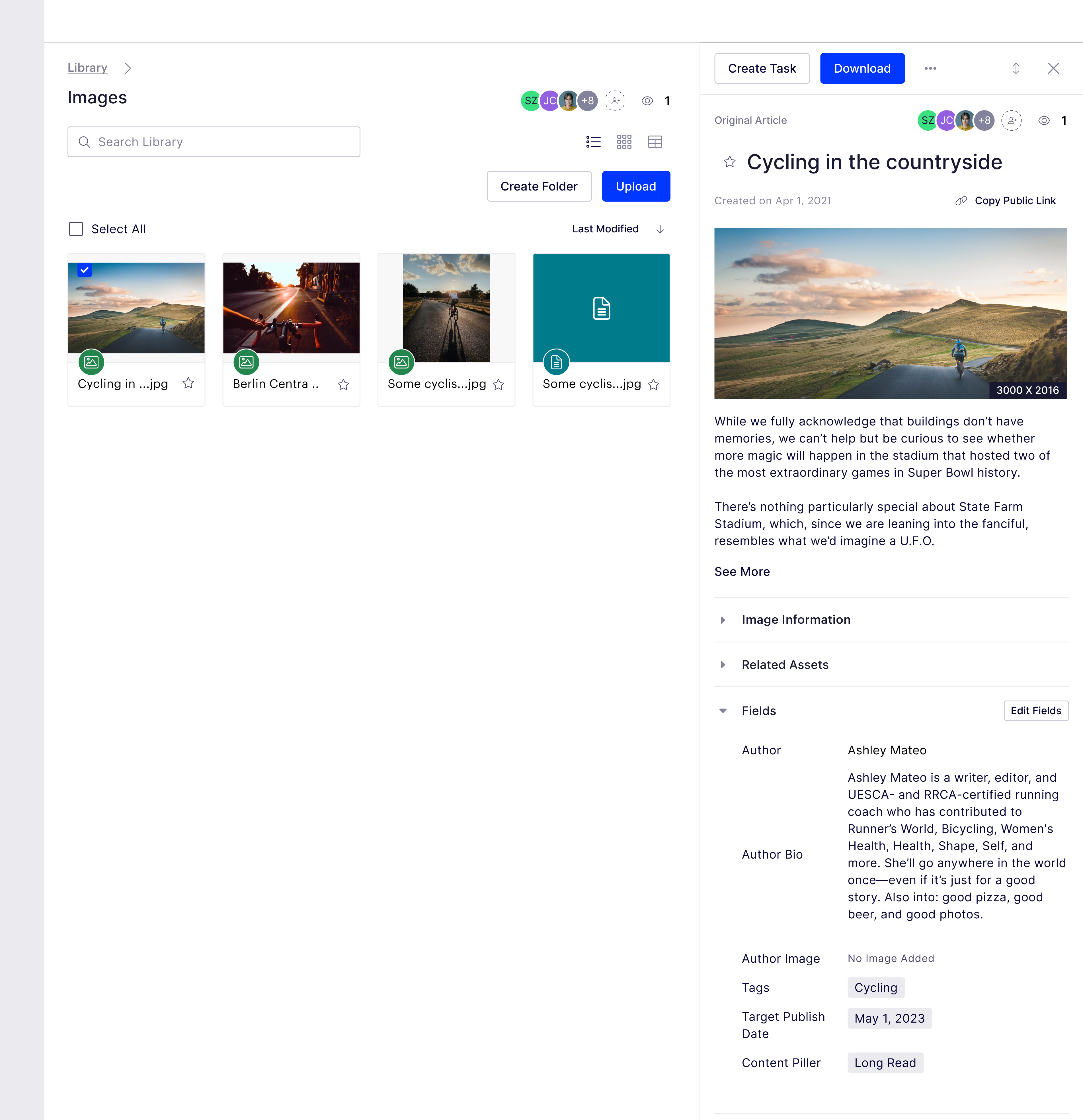This image shows a screenshot from what appears to be a photo or stock image website. The interface features a clean, white background. A gray vertical bar on the left spans from the top to the bottom of the screen. This left panel, occupying roughly two-thirds of the screen, contains a section titled "Library" followed by a display of images, likely resulting from a user search that yielded four results.

To the right, a column offers options for user interaction. At its top, buttons labeled "Download" and "Create Task" are visible. Beneath these buttons, the heading reads "Cycling in the Countryside," introducing the selected photograph.

Below the heading, a block of text intriguingly states, "While we fully acknowledge that buildings don't have memories, we can't help but be curious to see whether more magic will happen in the stadium that hosted two of the most extraordinary games in Super Bowl history."

Further down, detailed metadata about the image is available, including sections like "Image Information," "Related Assets," "Fields," "Author," "Author's Site," "Author Image," "Tags," and "Date Published," which is listed as May 1st, 2023. The content is categorized as a "Long Read."